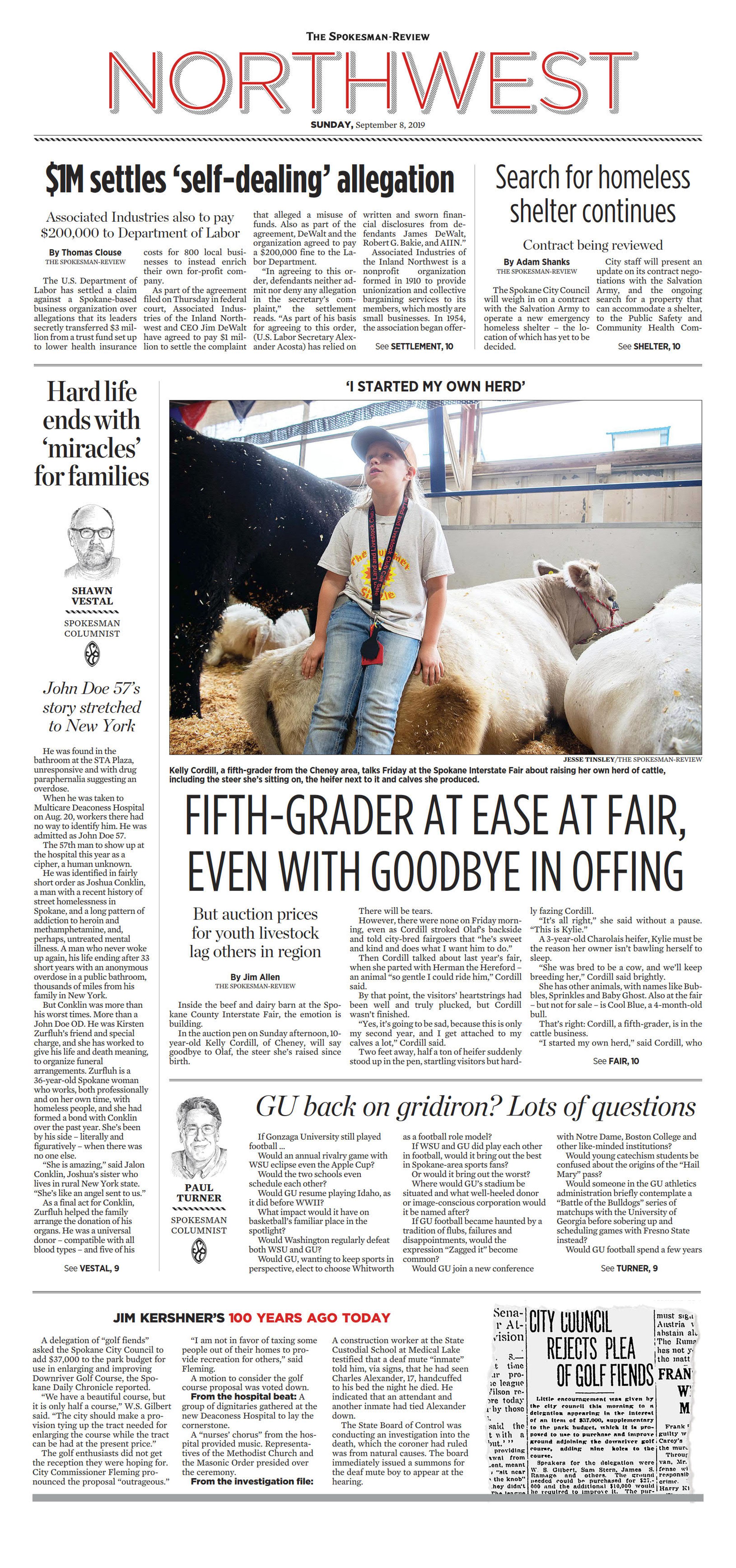This image is a blurred screenshot of a digitalized newspaper titled "The ***** Review Northwest." The exact edition is unreadable, and the word preceding "Review" is obscured.

The main headline is prominently featured:
- "**Fifth Grader at Ease at Fair, Even with Goodbye and Offing**" 
  - Accompanied by a photograph of a young child, likely around fifth grade age, leaning against a cow that is lying on the ground, with another cow beside them. The child, dressed in jeans, a t-shirt, and a baseball cap, appears to have a trophy around their neck. The caption above this image reads, "I Started My Own Herd."

Other noticeable headlines include:
- "**One Million Settles Self-Dealing Allegation**" 
- "**Search for Homeless Shelter Continues**" 
- "**Hard Life Ends with Miracles for Family**" 
  - This article is accompanied by a picture of a balding man wearing glasses.

Additional sections headline:
- "**GU Back on Gridiron, Lots of Questions**" 
- "**City Council Rejects Plea of Golf Friends or Fiends**"

The overall presentation of the newspaper hints at a range of community-centered stories covering local events, legal settlements, societal issues, sports questions, and more intimate human interest stories.